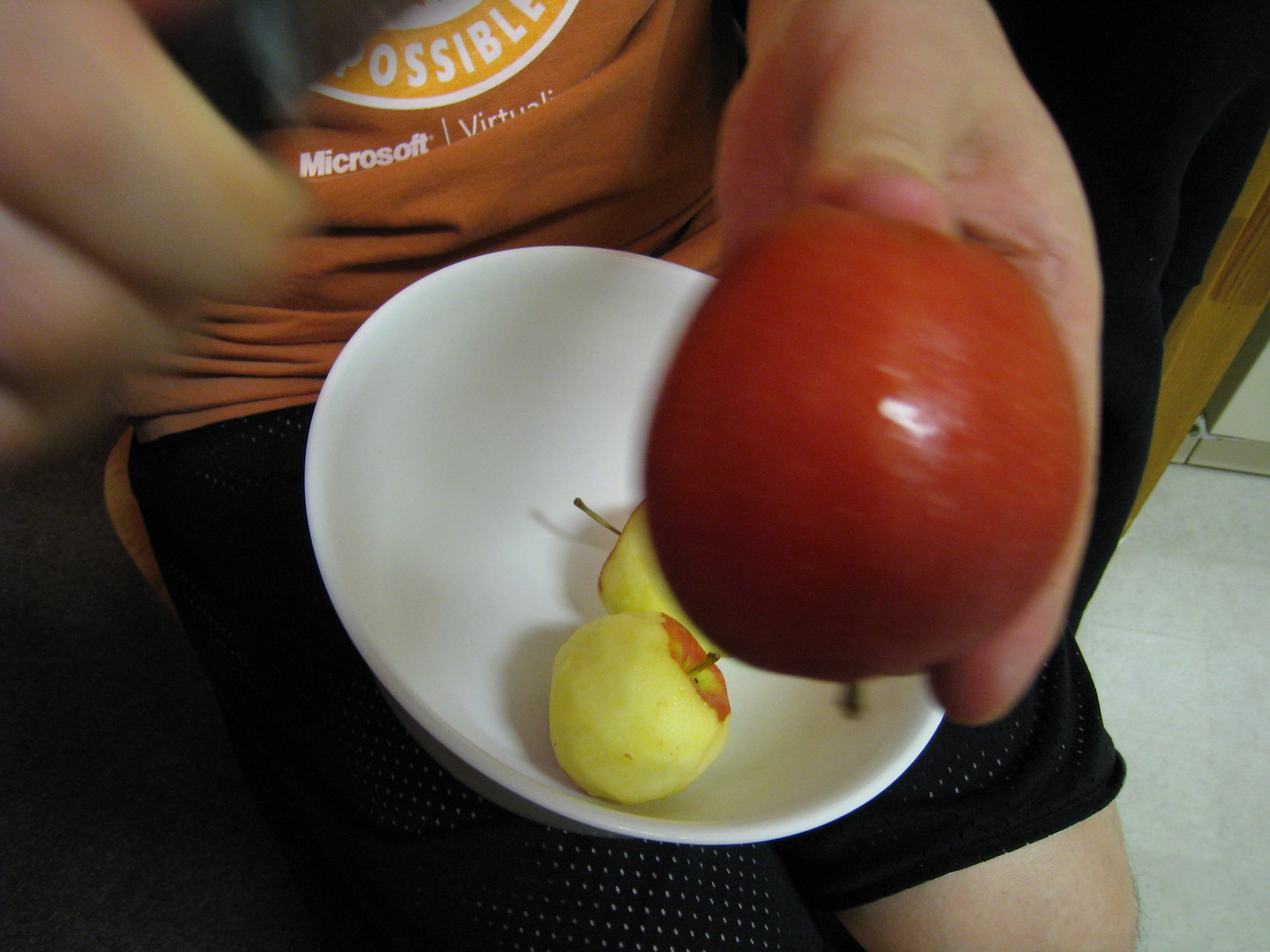In the image, a person is seated, wearing a rust-colored t-shirt with partial text that hints at the word "possible" and possibly something about "Microsoft" in white letters. They also wear black shorts flecked with white dots. The focal point of the scene is the person's hand, which holds a perfectly round, very red apple, displayed upside down with its stem at the bottom. In front of them, a white bowl contains two smaller, peeled apples with exposed flesh and just a hint of their original red skin near their stems. The setting features a simple grayish floor, and overall, the environment is nondescript and plain. The vivid red of the unpeeled apple, almost orange in hue, sharply contrasts with the more muted and natural tones of the rest of the scene.